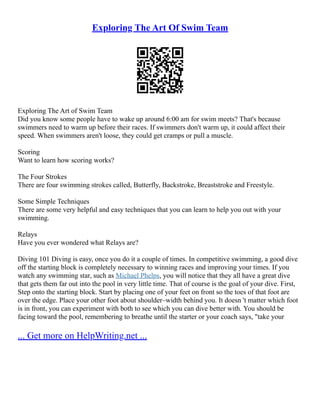The image features a screenshot of text with a detailed description titled "Exploring the Art of Swim Team" in blue and underlined, indicating a hyperlink. Below this is a QR code, followed by the same title in regular text. The main body of the text provides educational insights about swimming. It starts by highlighting that swimmers often wake up around 6 AM for meets to ensure they have time to warm up; failure to do so can negatively affect their speed, causing cramps or pulled muscles.

Further along, the text explains competitive swimming themes such as scoring, the four primary strokes (butterfly, backstroke, breaststroke, and freestyle), simple techniques to enhance swimming, and an introduction to relays. The final section, titled "Diving 101," emphasizes the importance of a strong dive off the starting block for winning races and improving times. It even includes a step-by-step guide for proper diving technique, mentioning the significance of a well-executed dive as demonstrated by swimming stars like Michael Phelps, who achieve significant distance quickly. The text stops abruptly with instructions to breathe until the starter or coach gives the cue. At the bottom, another piece of blue, underlined text directs readers to "get more on helpwriting.net." The entire document is presented on a white background and the font is very small.